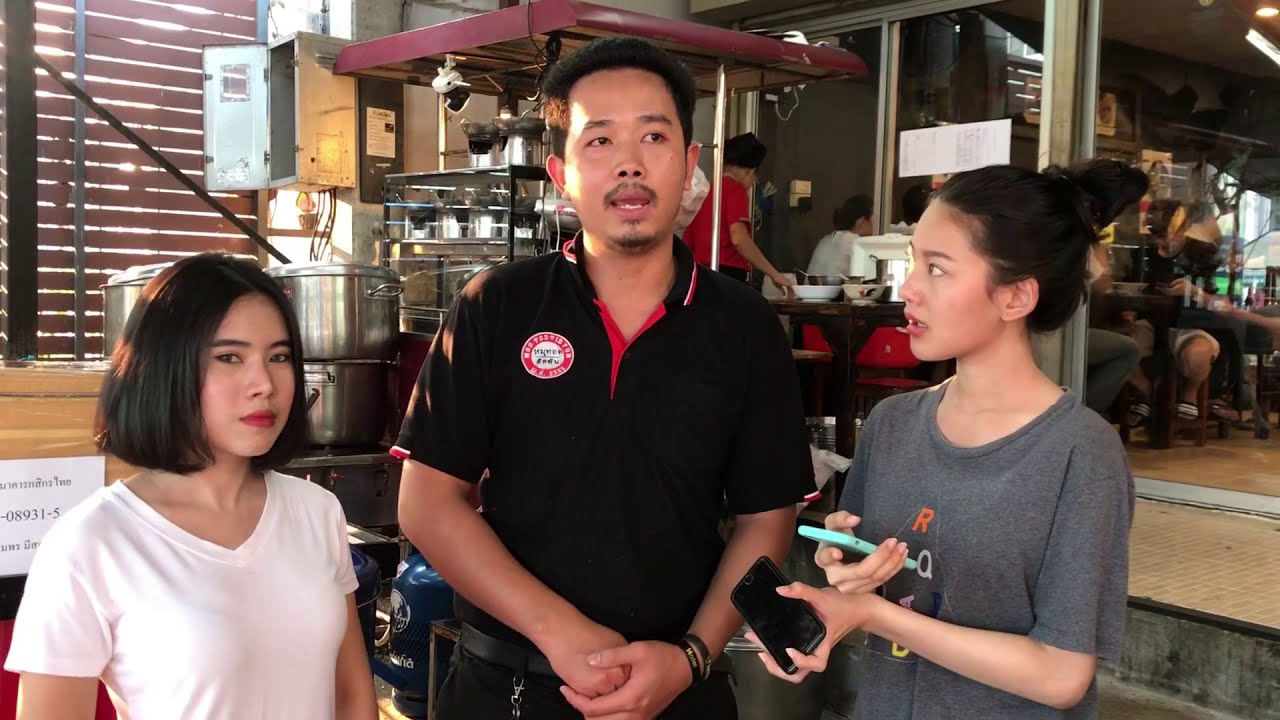In this brightly lit kitchen, sunlight filters through wooden blinds, casting a warm glow on the scene. Three young Asian individuals are the focal point, standing amidst an array of kitchen utensils like pans, glasses, and cups that hint at a bustling culinary environment. In the center stands a tall man with short hair and black facial hair, sporting a black short-sleeved shirt with red accents and an indistinct logo, paired with black slacks. He appears to be speaking, possibly being interviewed. To his right, a woman in a gray short-sleeved t-shirt with 'RQ' on it is holding a black and blue cell phone, likely recording him. On his left, another woman in a white V-neck short-sleeved t-shirt stands with a stern, solemn look directed at the camera. She is slightly shorter, with hair that catches the sunlight. Behind them, you can glimpse large window panes that stretch from floor to ceiling, revealing a dining area with people seated at tables, suggesting the kitchen is part of a restaurant.